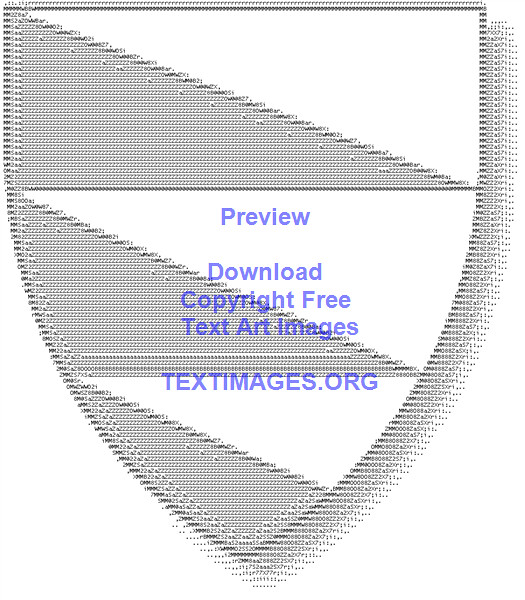The image is of a shield, characterized by a plain white backdrop and sections divided by three silver-colored triangles arranged from left to right. These triangles are long and jutting out, giving them a material-like, almost 3D appearance with intricate design patterns that add depth. A light-colored shadow surrounds the entire shield, enhancing the 3D effect with lighter grays and whites, contributing to a dotted, slightly dizzying visual.

In the central portion of the shield, there's a slightly right-justified watermark in light lavender, containing a series of words stacked vertically in blue text. It starts with "Preview" under the first triangle, followed by "Download," "Copyright Free," and "Text or Images." At the near-bottom edge in all capital letters, it says "TEXTIMAGES.ORG." Closer inspection reveals that the lines forming the image are composed of tiny numbers and letters, adding a textured, almost fuzzy look to the design.